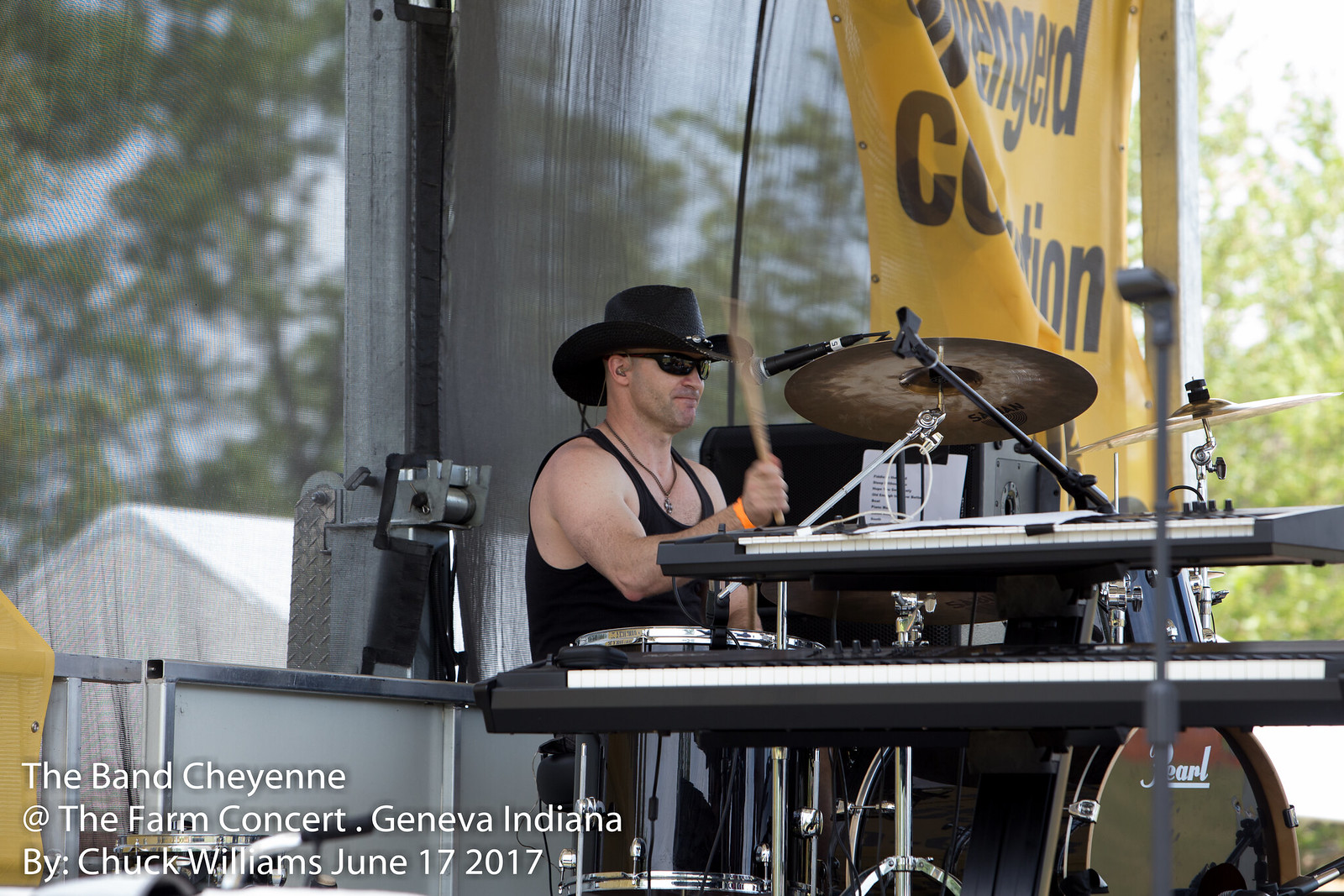A husky man, around 35 years old, is captured in mid-performance at a drum set, evidenced by the motion blur of the drumstick in his raised right hand. He dons a black cowboy hat, dark sunglasses, a dark necklace, and a black sleeveless T-shirt. An orange band adorns his right wrist. The stage is partly framed by keyboards that resemble piano keyboards in the foreground, while behind him, a gray curtain with an undecipherable yellow banner hangs. To his right, a white tent is visible, and a fence with trees can be seen on the horizon. In the lower left corner of the color photograph, which is in landscape orientation, white text reads "The Band Cheyenne at the Farm Concert, Geneva, Indiana by Chuck Williams, June 17th, 2017." The drum set in front of him is labeled with the Pearl brand.